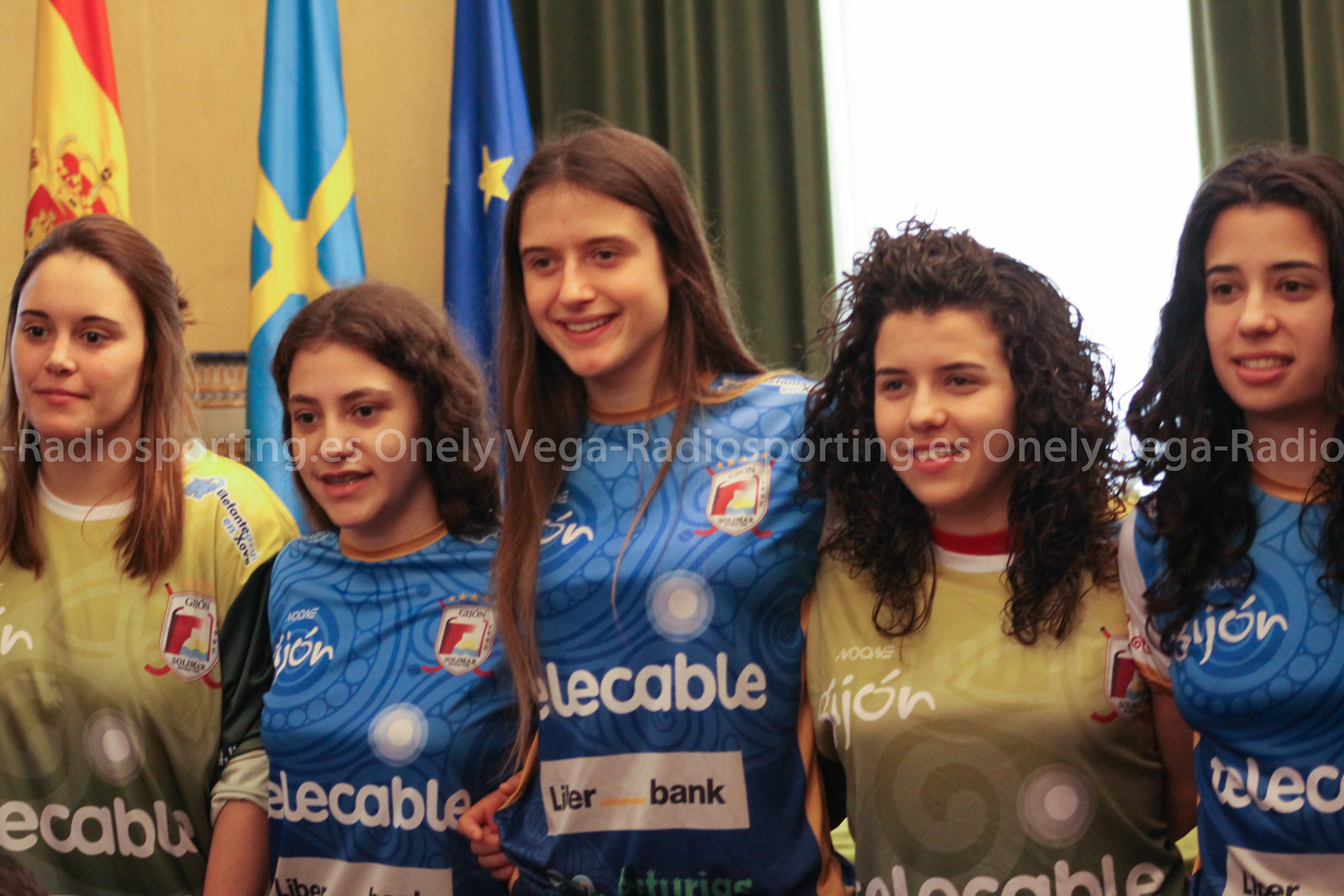This photograph features five young women, possibly in their late teens to early 20s, who are all members of the same team. They are wearing uniforms with jerseys that have various sponsors such as "Telecable," "Liar Bank," and "Elekabal" printed on them. The jerseys are predominantly blue for three of the women, while the remaining two wear a light green or yellowish-green shade. From left to right, their uniform colors follow the pattern: green, blue, blue, green, blue.

In the background, the setting appears quite official, featuring heavy green drapes and a window visible between them. There are also three flags, one of which is red and yellow, while the other two are blue with distinctive patterns - one with a yellow cross and the other with stars.

The women are standing close together, posing for the photo with smiles, suggesting a moment of celebration, possibly after a recent victory in a tournament. They all have their hair down and display a happy demeanor, clearly enjoying the moment. The caption "Radiosporting.es" and "Only Vega" watermark can be seen in the image.